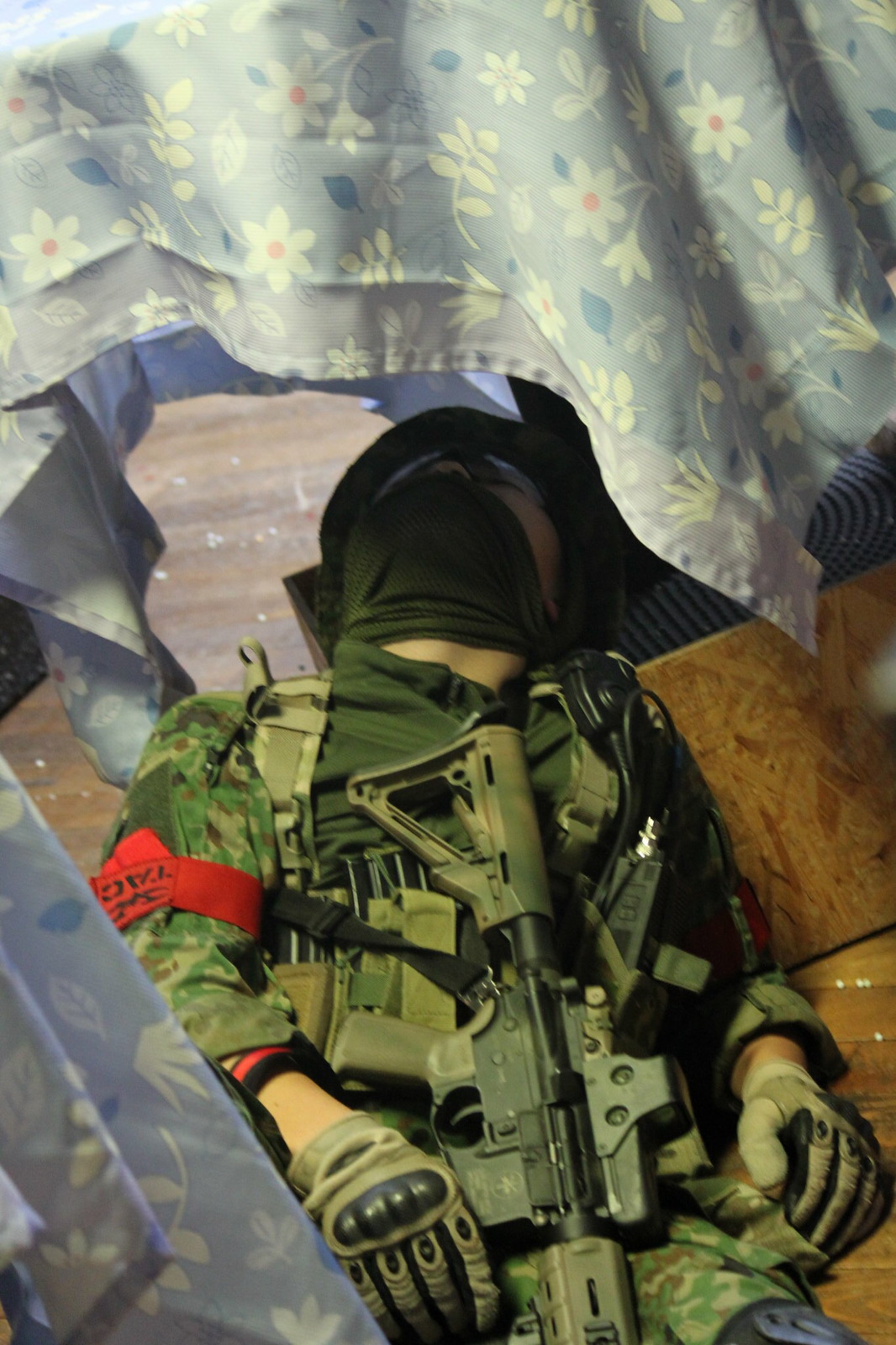A photograph captures a soldier lying prone on the ground, dressed in a camouflage outfit comprised of shades of dark green and brown. He wears green and black padded gloves, and a rifle with a metallic green finish, matching his camouflage, rests across his chest with the barrel pointed downward. A bright red band adorns his right arm, standing out vividly against the muted tones of his uniform. His face is partially obscured by a green face covering that conceals his chin. Above him, a piece of blue fabric decorated with white flowers adds a contrasting splash of color to the scene.